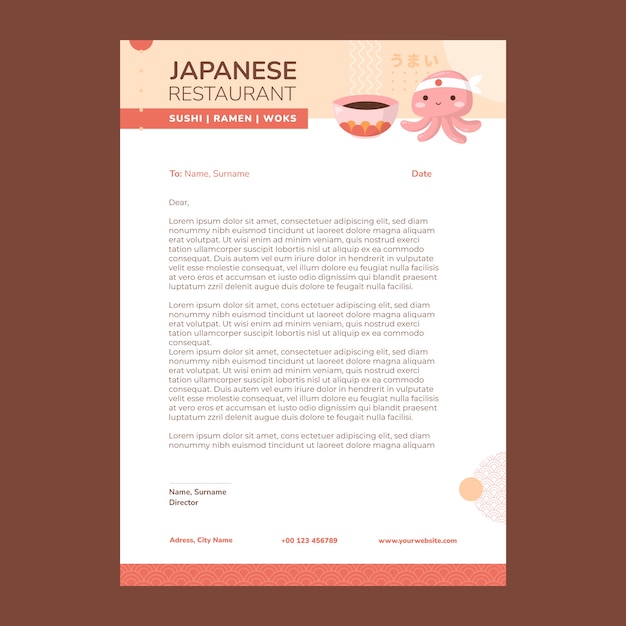The image is a digital mockup of an 8.5 by 11 flyer for a Japanese restaurant, crafted with a playful border featuring a cute pink octopus or squid sporting a white headband adorned with a Japanese star and circle. At the top of the flyer, the restaurant's specialties – "sushi, ramen, walks" – are prominently displayed. The central area of the flyer serves as a template letter that begins with placeholders for a recipient's name, surname, and date. The letter starts with "Dear," followed by two paragraphs filled with placeholder text like "lorem ipsum.” It concludes with "Name Surname, Director" and includes blank spaces for the restaurant's address, phone number, and a generic website URL, "yourwebsite.com," at the bottom. Additionally, the octopus is depicted smiling beside a hot bowl of soup or tea, adding an engaging visual element to the minimalistic letterhead design.